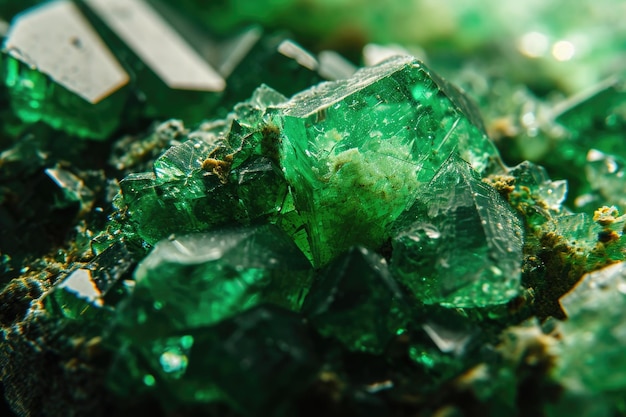The photograph showcases a detailed close-up of a green, rough-cut gemstone, possibly an emerald or jade, prominently situated at the center. The main crystal, which is wider at the bottom and narrows towards the top, exhibits a somewhat murky interior, suggesting potential impurities. Surrounding this central piece are various smaller, jagged stones scattered on the ground, with shapes resembling pyramids and tombstones. These additional crystals are slightly out of focus, hinting they are part of the same natural environment, possibly a mining site. The setting appears to be earthy, with patches of yellow moss dotting the area around the stones. The background displays more of these green gemstones, but they are blurred, emphasizing the principal crystal at the center of the composition.